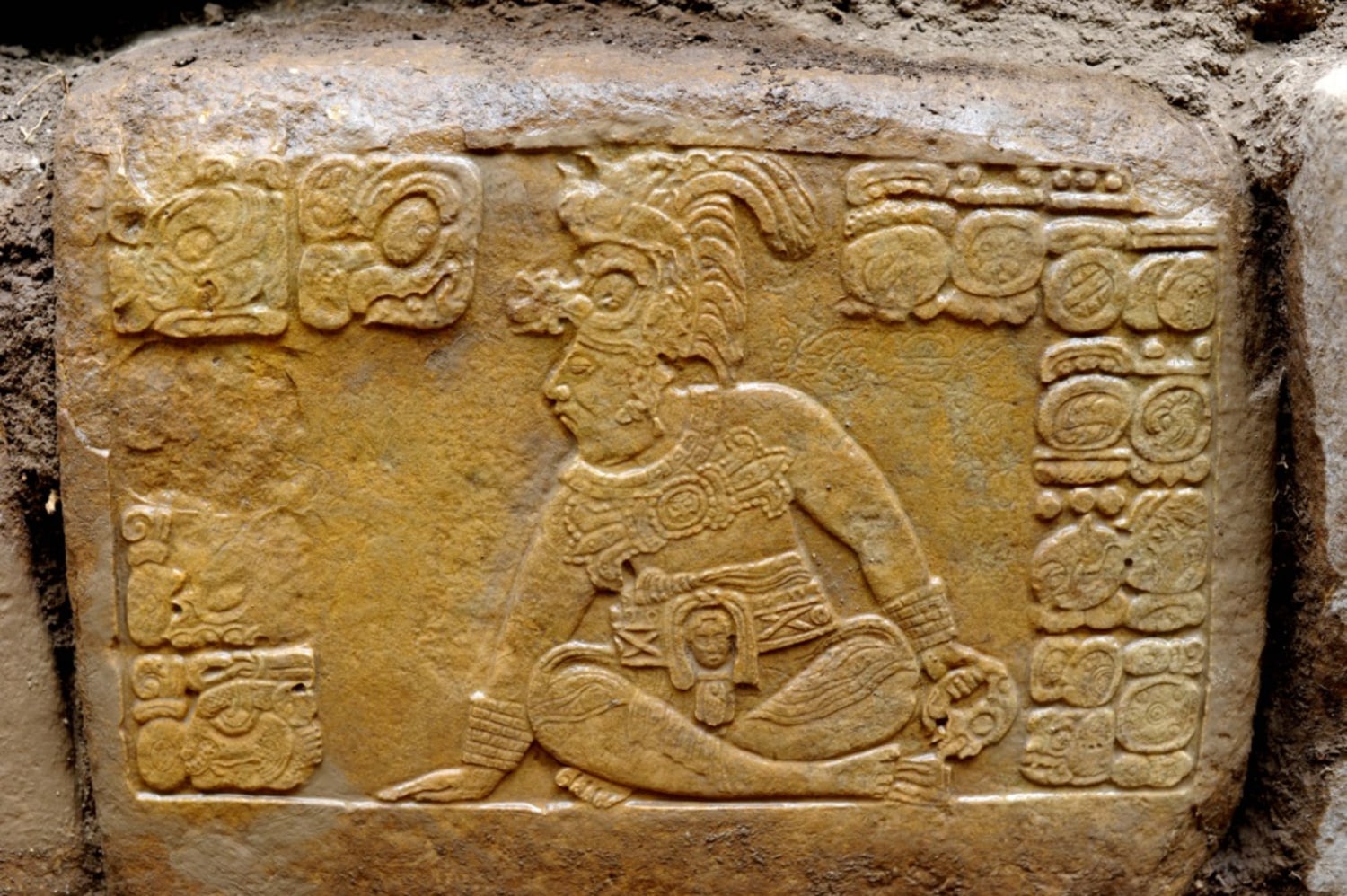The image depicts a detailed carving on a yellow stone, likely from the Aztec or Mayan era. At the center of the stone, a man is depicted sitting with his legs crossed, adorned in cultural attire including animal-type headgear and a garment around his waist. The man is facing left. Surrounding the central figure are uniquely designed squares or tiles, some resembling faces or animal heads. The top of the stone is a very chiseled gray, with pieces of debris scattered across it. The stone appears to be part of a larger structure, although the image is focused exclusively on this single carved section.